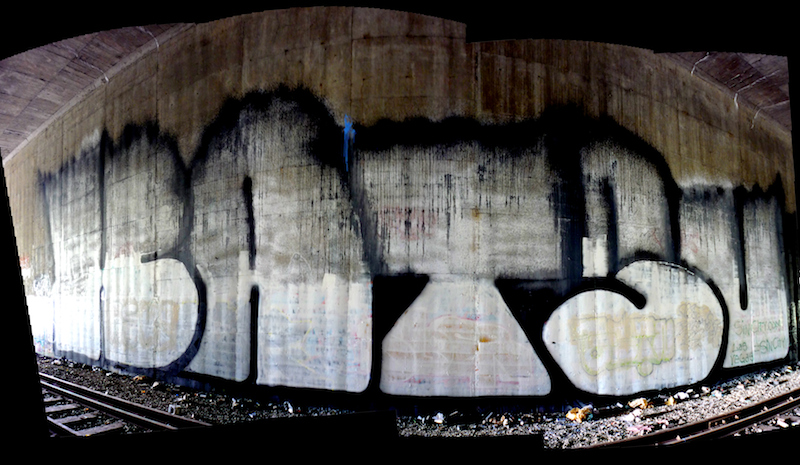This image is a composite photograph of a graffiti-tagged wall next to a railroad track, likely taken in a train tunnel or subway underpass. The image appears to be a panoramic shot, comprised of multiple photos pieced together, as evidenced by the curved edges and noticeable photo seams. The graffiti prominently displays large, stylized bubble letters that spell out "Ibahtsu" or "BATSU," in white with a black outline. The wall itself is concrete, dirty, and grungy, with various signs of wear, tear, and moisture damage. The scene is littered with trash, adding to the overall gritty atmosphere. Train tracks are visible in the lower left and right corners, distorted at improbable angles due to the likely use of a wide-angle or fisheye lens. The background is predominantly dark, enhancing the stark contrast of the graffiti on the wall.